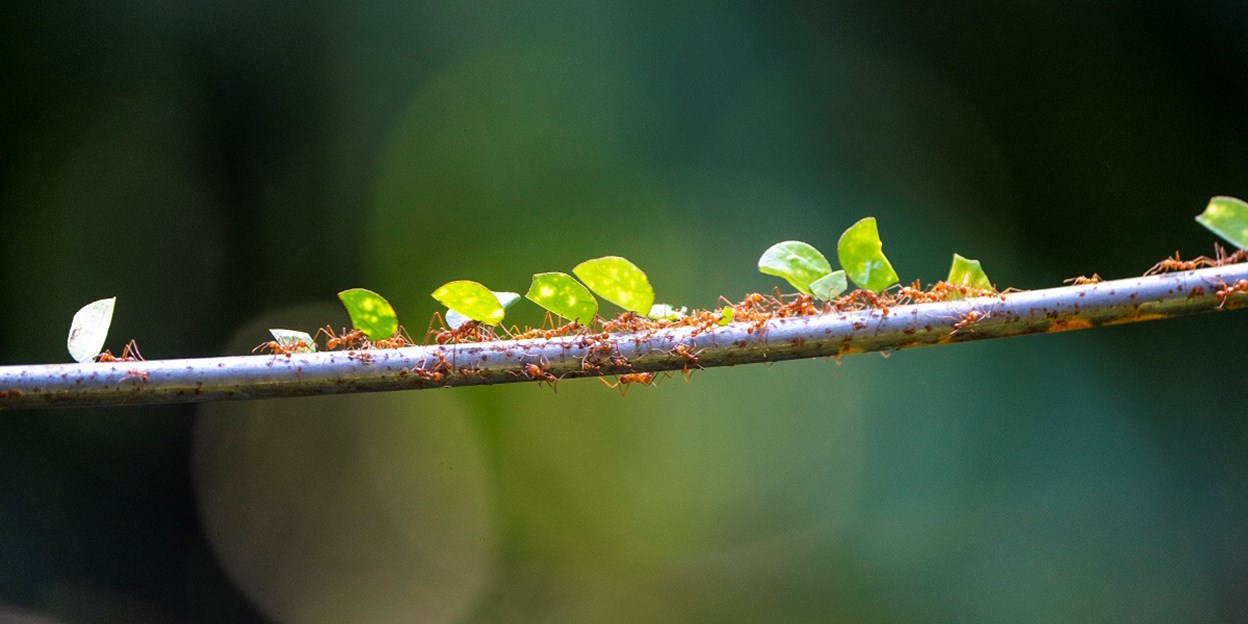This detailed wildlife photograph captures a vivid scene of red ants diligently working on a branch that spans horizontally across the image from left to right. The background is a blurry mix of green, bluish, and yellow hues, likely suggesting a forest or nature setting, but remains indistinct to highlight the ants in sharp focus. The centerpiece of the picture is a somewhat rusty branch or twig, heavily populated with red ants. The ants are seen busily crawling along the branch, with many of them carrying green leaves, some dotted with yellow. Their coordinated march primarily appears to be from right to left, showcasing the ants' remarkable organization and effort in transporting the leaves. Several ants are also clinging to the underside of the branch, adding to the dynamic sense of activity within this bustling miniature world.